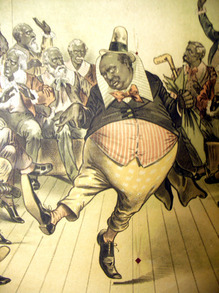The illustration is an antique piece, likely dating back to the 1800s, evidenced by its aged, yellowed appearance with a beige sepia tone that suggests it's been affected by time. Dominating the scene is a rotund, black-skinned man with ambiguity surrounding his skin tone due to the peculiar coloring that suggests either discoloration over time or intentional artistic choice. He sports a small, thin, black and white hat perched atop his round head, and he's clad in an ill-fitting black morning jacket. His outfit is complemented by a large white collar, a bright red bow tie, and a red and white striped vest that spills over his substantial pot belly. His ostentatiously yellow pants are adorned with white spots, and his shoes are exaggeratedly long and thin. In his hand, he holds an umbrella, implying he's engaged in a whimsical dance on what appears to be a wooden floor. Surrounding him are several African-American men with gray skin and white facial hair, all attired in formal wear. These men, seemingly a jazz band or a group of musicians, are either engaged in animated conversation or playing instruments, paying little heed to the dancing man in their midst. The overall scene exudes a surreal, almost caricatured atmosphere, marked by the peculiarities of its coloring and the exaggerated features of its characters.